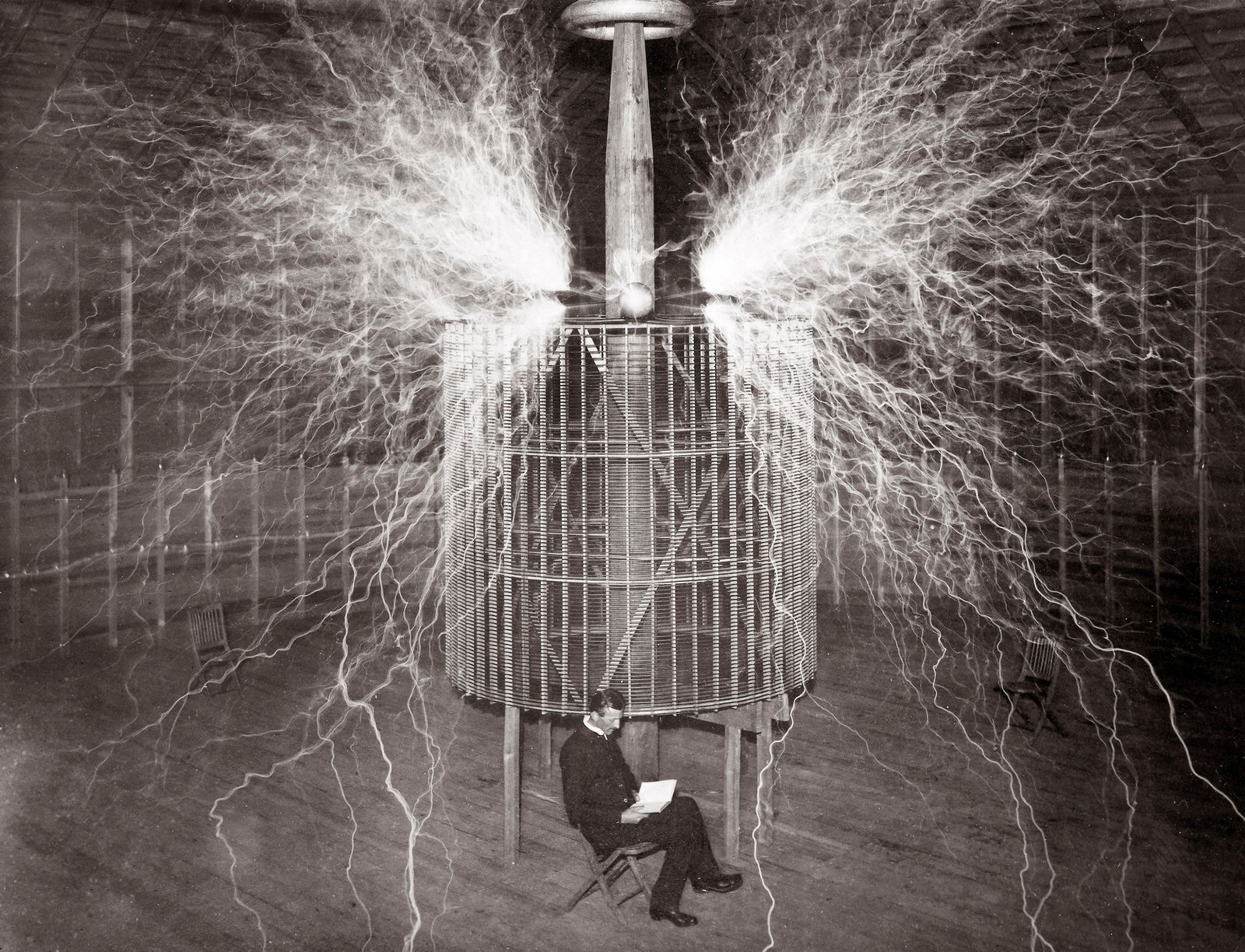This black and white photograph captures a tall man, who is very likely Nikola Tesla, seated in a large, vintage room that appears to be one of his famous electricity power plants. The man, dressed in a black suit with a small white collar, sits in a small wooden chair with a book open on his lap, seemingly absorbed in his reading and unfazed by his surroundings. His legs are crossed, and he has short hair. Behind him stands a large cylindrical apparatus, resembling a Tesla coil, made of metal with a central pole and a spherical top. This device is emitting intense streams of electricity in all directions, creating a dramatic and intricate display of electrical sparks that look like lightning or spider-web-like veins. The floor of the room appears to be wooden, adding to the vintage atmosphere of the photograph.